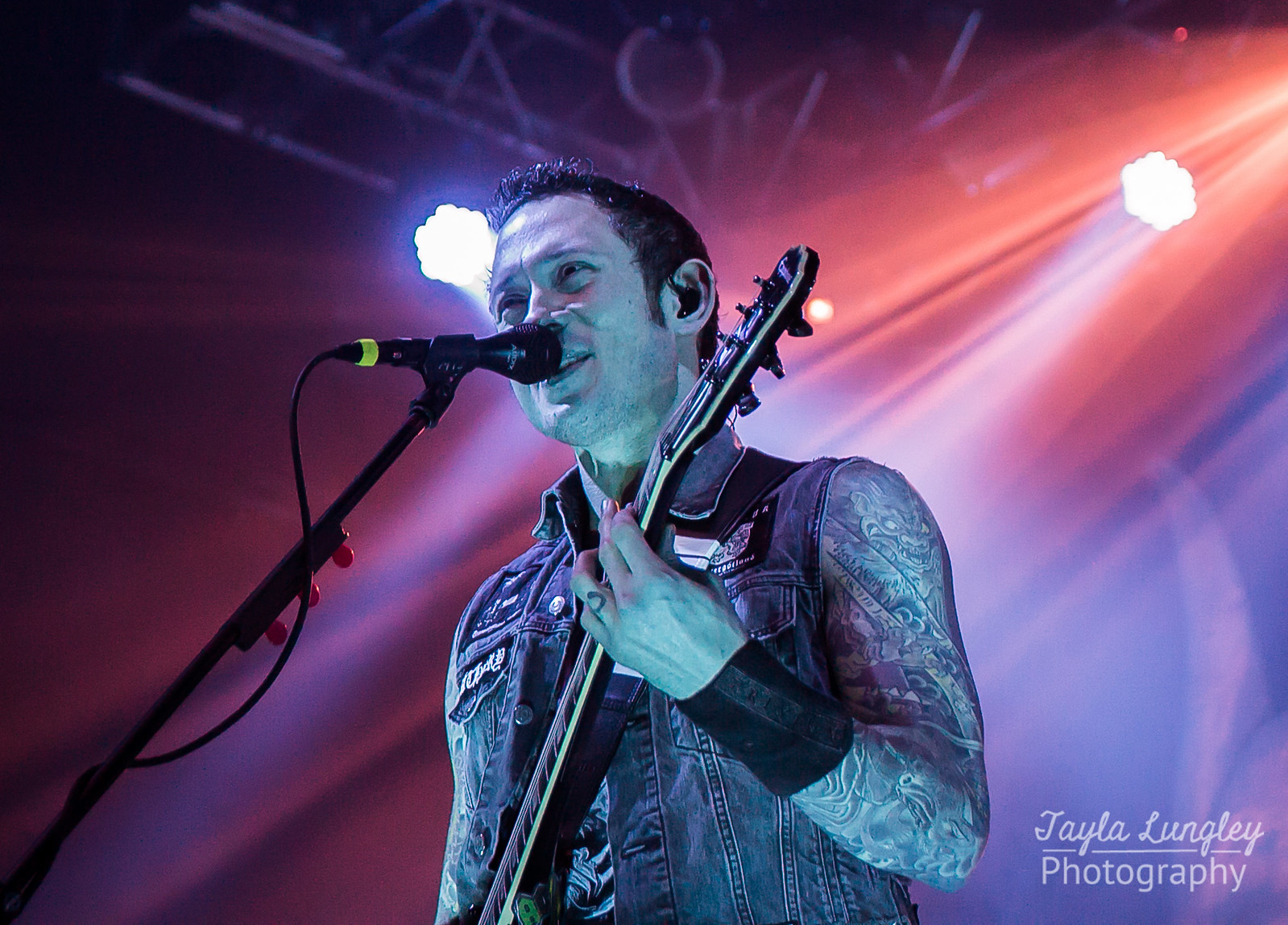This is an image of a young white man, a musician performing live on stage, captured by Tayla Lungley Photography. The scene features him singing into a microphone attached to a mic stand adorned with three red guitar picks and a yellow band. He is playing a black electric guitar, supported by a strap around his chest. The musician is wearing a blue, faded, sleeveless jean vest, resembling a Levi's jacket, and has numerous tattoos covering his arms from his shoulders to his wrists. His short black hair is gelled, and he is using in-ear monitors. A black wrist support is visible on his left wrist, which is positioned on the guitar neck. The stage setup includes scaffolding in the background, rigged with white and yellow spotlights that cast a dramatic glow behind him. The overall ambiance of the performance area is dimly lit, accentuating the focused light on the musician.